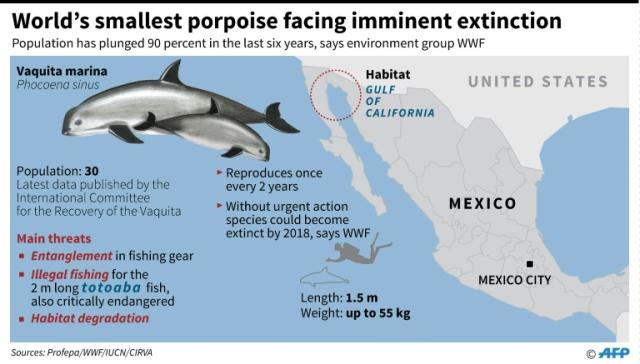This detailed infographic, entitled "World's Smallest Porpoise Facing Imminent Extinction," highlights the critical endangerment of the Vaquita Marina (scientifically known as Phocoena sinus). The poster, predominantly blue with a white header, displays the alarming statistic that the population of these porpoises has plunged 90% over the last six years according to the WWF. Current population estimates by the International Committee for the Recovery of the Vaquita show only 30 individuals remain as of the latest data. The main threats to their survival include entanglement in fishing gear, illegal fishing for the critically endangered Totoaba fish, and habitat degradation. The infographic also notes these porpoises reproduce only once every two years, warning that without urgent action, they could have become extinct as early as 2018. An illustration of the Vaquita Marina showcases their silvery bodies, blunt heads, and distinctive black fins and tails. Additionally, a map highlighting the Gulf of California area in Mexico, where these porpoises are primarily found, provides geographical context.